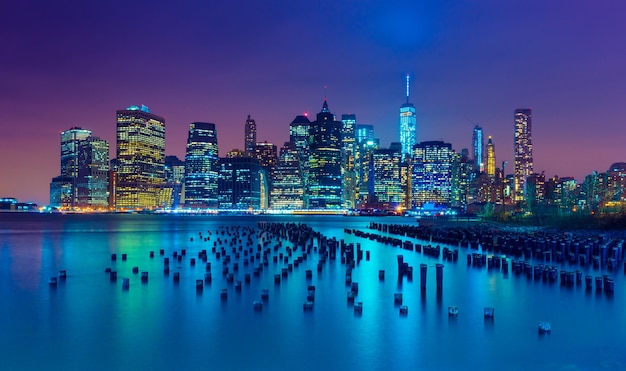This captivating nighttime cityscape photograph showcases a bustling metropolitan skyline adorned with plethora of illuminated skyscrapers and high-rise buildings. Dominating the right side of the image is a prominent tall building crowned with a spire, glowing vividly in blue. The city's lights, predominantly golden and blue, cast a mesmerizing glow against the backdrop of a purple and dark blue sky tinged with lighter pink and orange hues near the horizon. In the foreground, a tranquil body of water, possibly a river or bay, lies before the cityscape, reflecting the scintillating lights of the skyscrapers. This body of water is dotted with numerous wooden posts, creating an intriguing pattern of black dots and lines. The scene, rich in color and detail, effectively captures the vibrant essence of urban life at night.